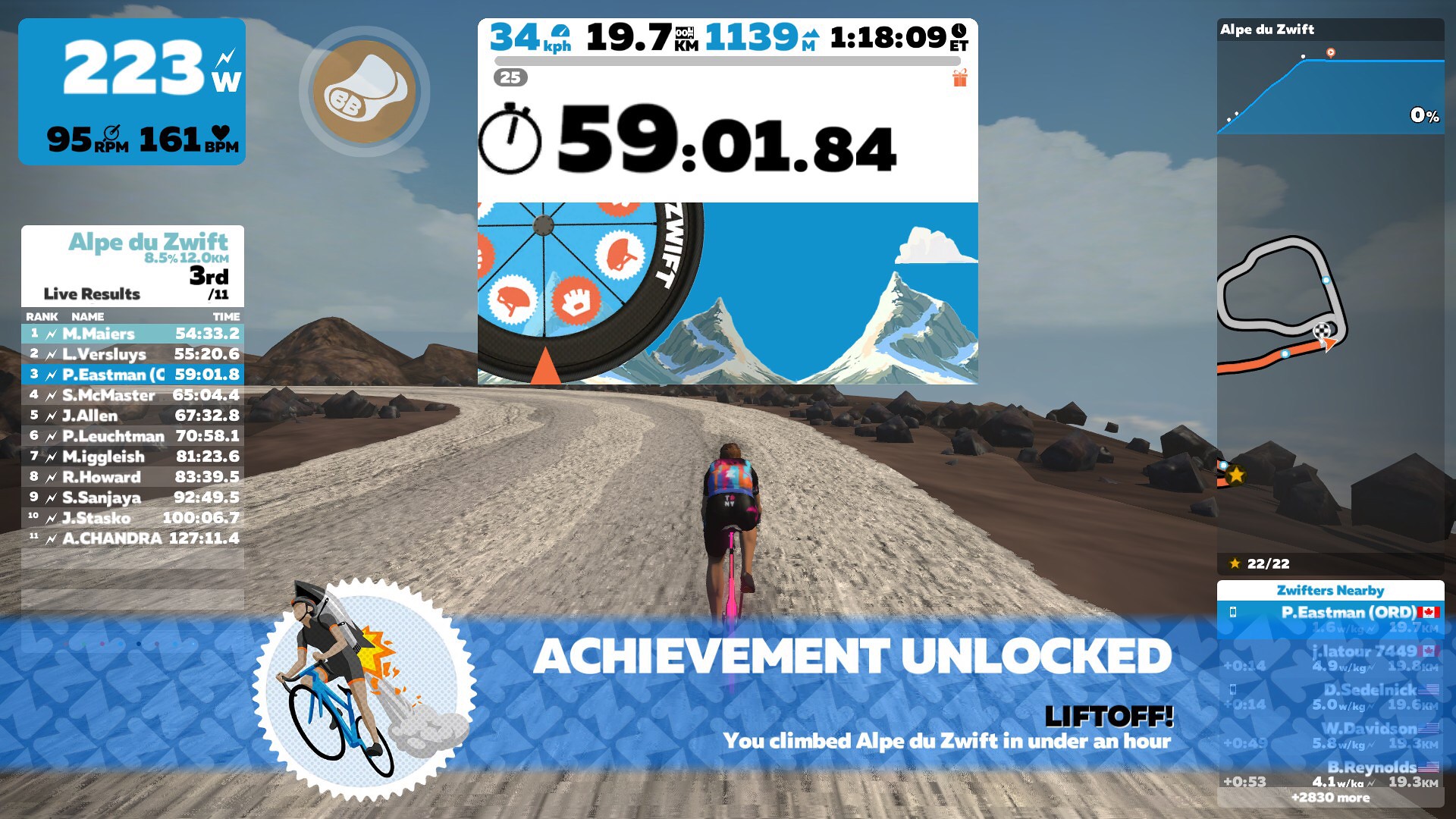The image appears to be from a virtual cycling game or an exercise program, possibly similar to Peloton or Zwift, featuring a colorful and dynamic scene. At the center, a person in black shorts and a multicolored top is depicted riding a bicycle on a gravel trail. Notably, there's an on-screen overlay providing various stats: the elapsed time (59:01.84), speed (34 kph), distance (19.7 km), elevation (1139 meters), and heart rate (161 bpm). To the left, power output is displayed at 223 watts, with a cadence of 95 RPM, and a leaderboard showcasing other participants. In the bottom section, a message in white bold text announces "Achievement Unlocked: You climbed up a Dude Swift in under an hour." The overall scene is vibrant with shades of blue, surrounded by brown mountains and gray rocks, under a clear sky. A small character on a bicycle with a rocket attached to it can also be seen on the left, adding a playful element to the image.